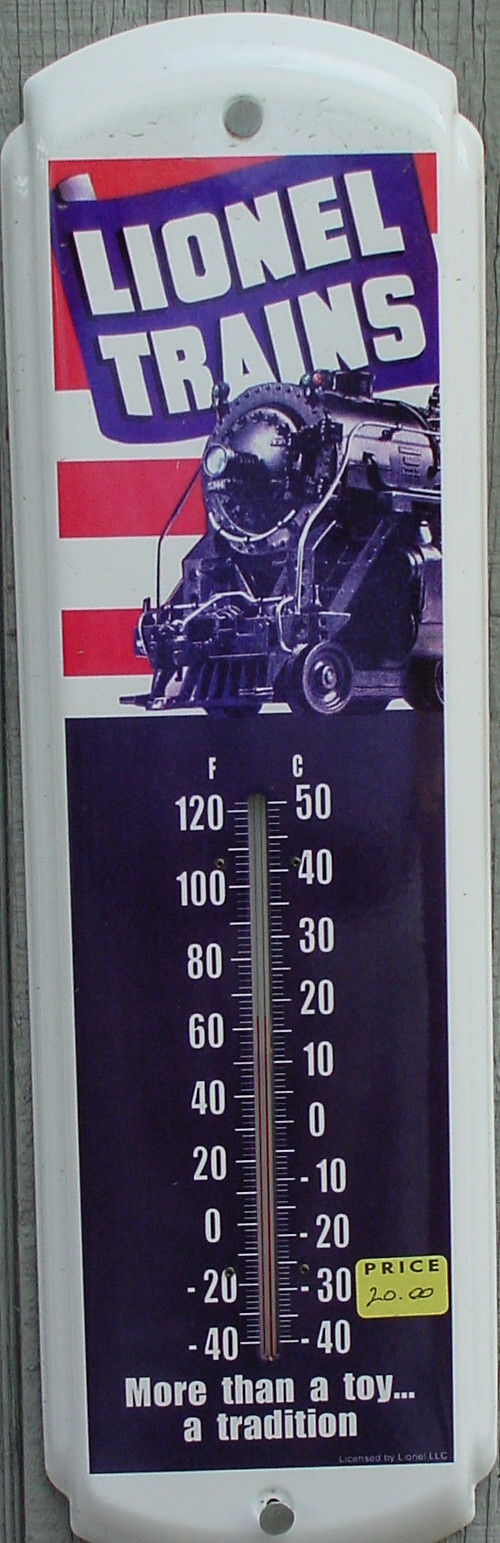**Detailed Caption:**

This photograph showcases a vintage wall thermometer with a nostalgic design. The thermometer is long and rectangular, crafted from metal with a white frame that adds a classic touch. Prominently displayed at the top is the iconic "Lionel Trains" logo, featuring a vibrant blue background with bold white lettering. In the center of this logo, there is an image of an antique steam locomotive, set against a red and white backdrop that highlights its timeless appeal. 

The thermometer itself features a dual temperature scale. The left side displays readings from -40 to 50 degrees Celsius, while the right side shows temperatures ranging from -40 to 120 degrees Fahrenheit. Both scales are marked with white numbers and tick marks on a striking black rectangular background, offering clear and precise readings.

At the bottom of the thermometer, inscribed in white lettering, is the phrase "More than a toy... a tradition," suggesting the long-standing heritage and cherished memories associated with Lionel Trains. For easy mounting, there are pre-drilled holes at both the top and bottom of the thermometer. Additionally, a yellow tag affixed to the lower right corner indicates the price, handwritten as $20, hinting at its collectible value.